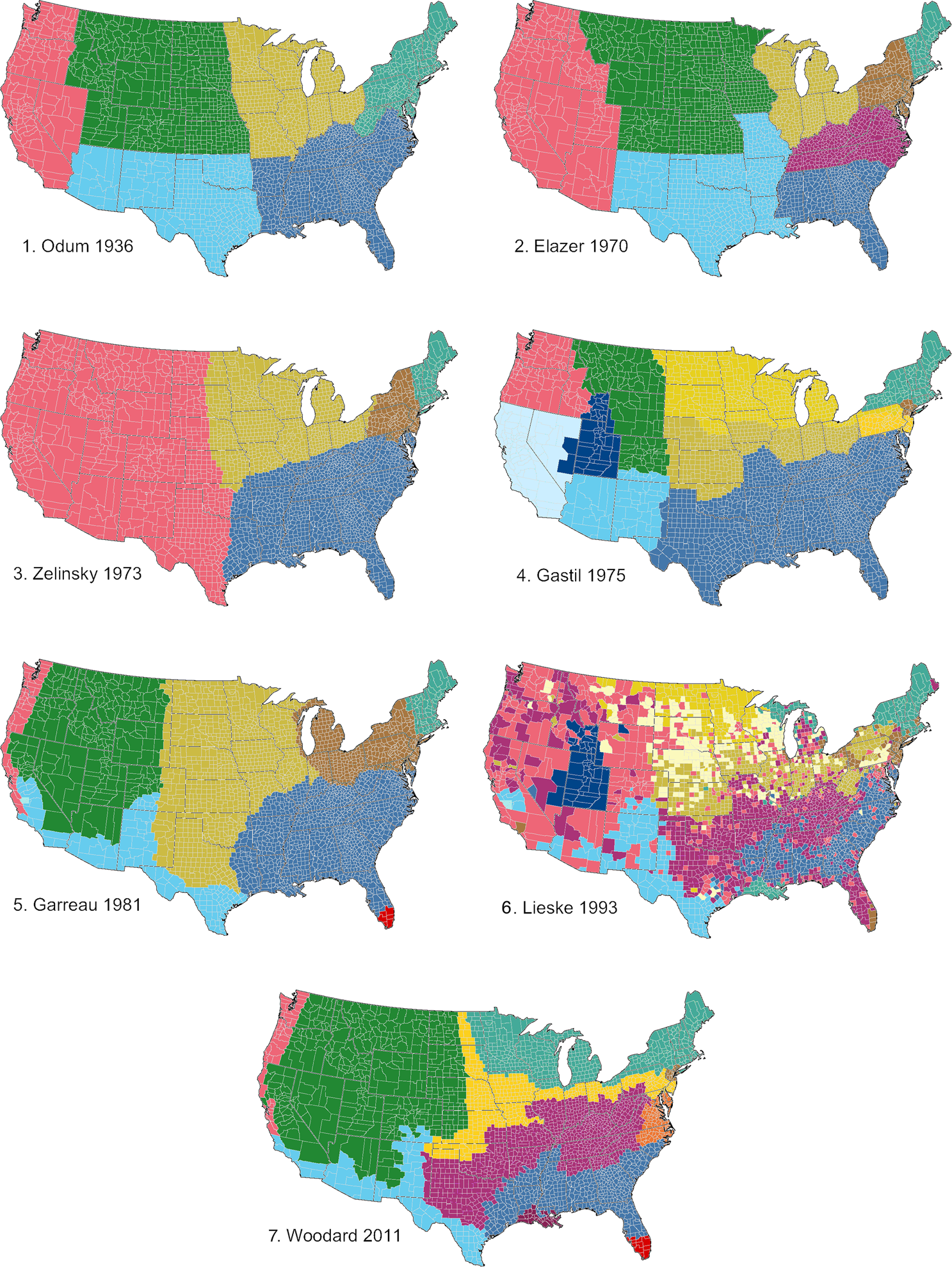The image displays seven vertically-aligned, rectangular maps of the continental United States, each distinctly color-coded to reflect geographical areas. These maps, arranged chronologically, provide a visual representation of shifting regional patterns over time. Each map bears a unique name and a specific year: the first map is labeled "Odium, 1936," highlighting California, Washington, Oregon, and Nevada in pink, the Northern Central U.S. in green, the Midwest in tan, the Southeast in blue, and the Northeast in teal. Subsequent maps—"Eliza, 1970," "Zielinski, 1973," "Gates, 1975," "Renault, 1981," "Lasky, 1993," and "Woodward, 2011"—show changes in these color-coded regions, suggesting demographic or environmental shifts over the years. Notably, the pink area expands in the Eliza map of 1970, while the blue regions along the East Coast diminish, indicative of these evolving patterns.